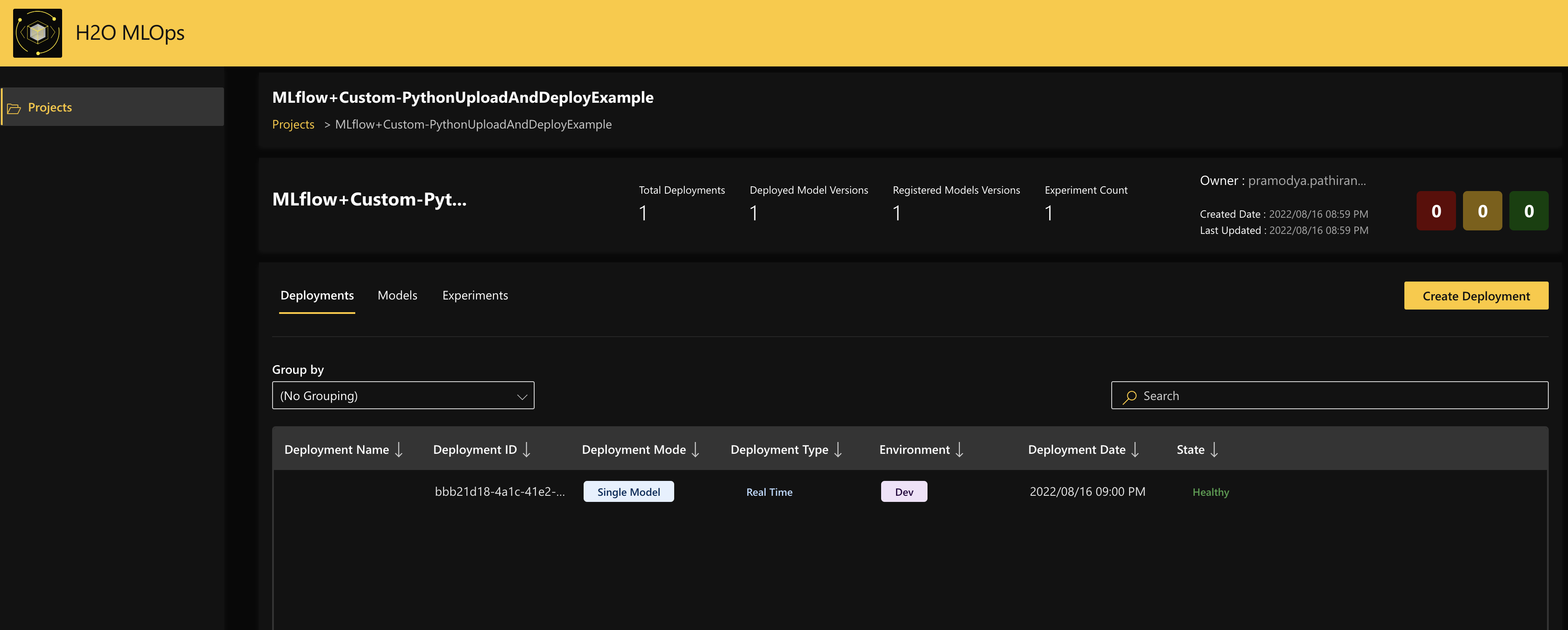### Detailed Caption for Screen Capture

The image is a screen capture of a monitor displaying a two-tone interface, predominantly featuring a vivid yellow banner across the entire top and a black window below it. In the top left corner of the yellow banner, there is a black square outlined with a yellow circle, inside which sits a white cube. To the right of this icon, black lettering reads "H2O MLOPS."

Underneath this section, on the left side, there is a lighter black bar displaying an open yellow file folder icon with the label "Projects" in yellow text next to it. On the right side of this black bar, there is white text against the jet-black background, stating "ML flow plus custom dash Python upload and deploy example." Directly below this, in yellow text, is another "Projects" label. Further down, there are more details related to ML flow and custom Python. This section includes statistics such as "Total deployments: 1," "Deployed model versions: 1," "Registered models versions: 1," and "Experiment count: 1," followed by "Owner: Pramodya Pathiran," though the information trails off the screen. Additional metadata mentions "Created date: 2022" and "Last updated: 2022."

Three square buttons are visible beneath this information, colored maroon, tan, and green, respectively. Below these buttons is a yellow bar labeled "Create Deployment," and further down is a search bar with a yellow magnifying glass icon. At the very bottom of the screen, a menu layout lists various groups both horizontally and vertically. The labels include "Deployment Name," "Deployment ID," "Deployment Mode," "Deployment Type," "Environment," "Deployment Date," and "State."